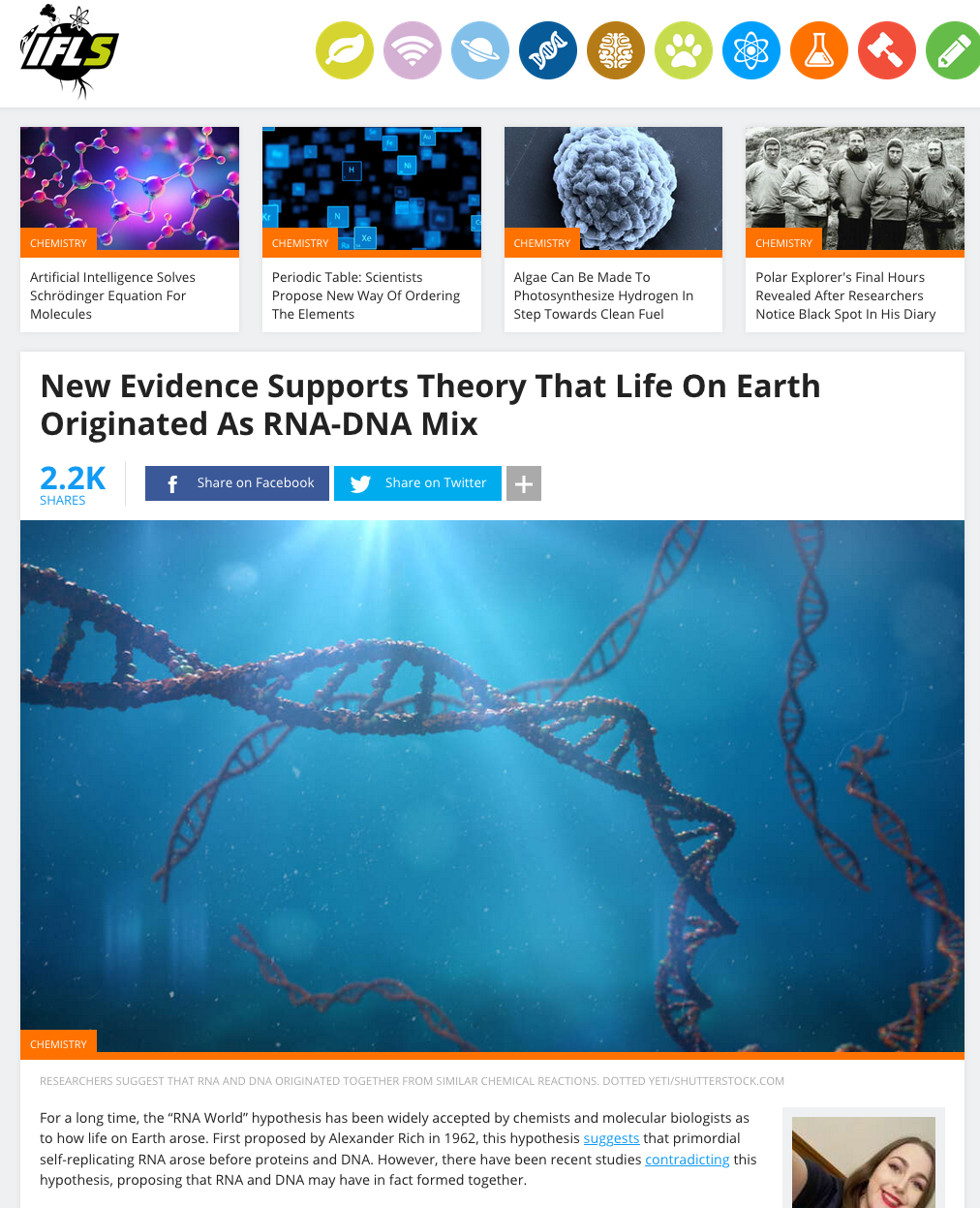The image depicts the home page of a niche science news website called IFLS. In the top left corner, the logo is prominently displayed, featuring the letters "IF" and "L" in white text, while the "S" is in green. The logo is overlaid on an illustration that appears to be a planet, likely Earth, surrounded by varied scientific symbols such as an atom and possibly some plant imagery, though the exact details are somewhat unclear.

At the top right of the screen, a series of thematic icons are aligned, representing various scientific disciplines. These icons include a leaf, Wi-Fi symbol, Saturn, DNA helix, tree, paw print, atom, beaker, gavel, and pencil, indicating a broad array of topics covered by the website.

Centralized at the top of the page, four headline articles are showcased. The topics of these articles are:
1. "Artificial intelligence solves Schrödinger equation for molecules."
2. "Periodic table: Scientists propose new way of ordering the elements."
3. "Algae can be made to photosynthesize hydrogen in step towards clean fuel."
4. "Polar explorer's final hours revealed after researchers notice black spot in his diary."

The most prominently featured article in the center of the screenshot highlights a groundbreaking study with the headline: "New evidence supports theory that life on Earth originated as RNA-DNA mix." This article appears to be the focal point of the current news cycle on the website.